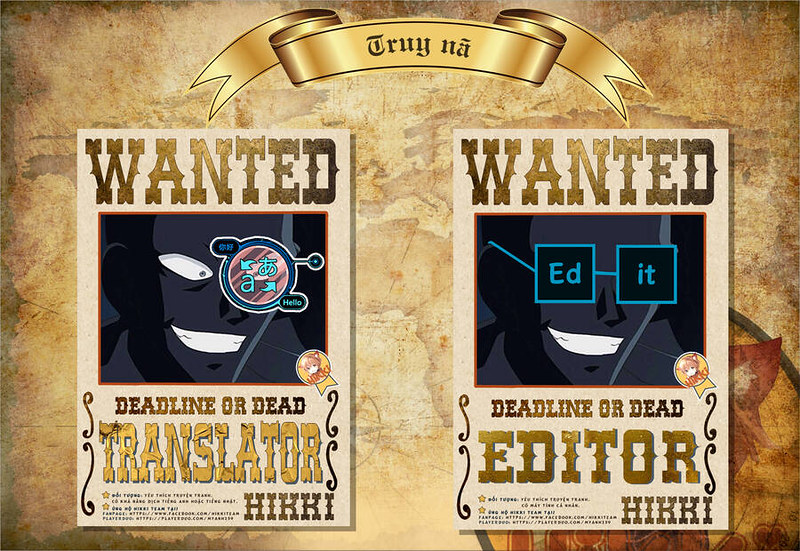The image is a detailed poster featuring a decorative gold scroll at the top, inscribed with the phrase "Truy Na" in an elaborate, illuminated manuscript-style font. Directly below the scroll are two side-by-side cartoon-esque wanted posters against a brown, parchment-like background, evoking an olden days aesthetic.

On the left poster, under the bold heading "WANTED," is the subtitle "Deadline or Dead Translator." The anime-styled character in the image has a monocle over his left eye, displaying random characters that represent translation, reinforcing the theme of language and translation tasks. Beneath this image, there is some small, unreadable text.

The right poster, similarly headed with "WANTED," reads "Deadline or Dead Editor." It features the same anime character, but this time he is wearing glasses with the letters "E.D." on the left lens and "I.T." on the right, symbolizing the editing process. This poster also contains some small, unreadable text at the bottom. The entire design speaks to a digital age representation of translator and editor roles through whimsical and artistic imagery.